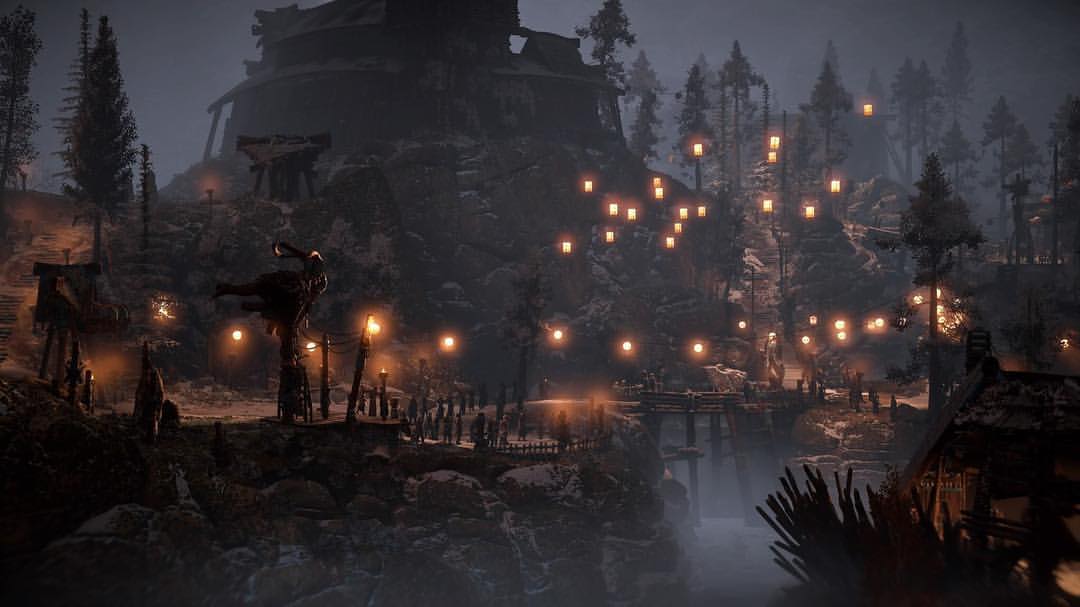The image is a captivating art piece depicting a dark, misty, and foggy mountainous village area, with a slightly snow-dusted, rocky terrain. It features tall trees scattered throughout, leading up to a prominent rocky cliff that hosts a large, boulder-like wooden building. The scene is illuminated by numerous large lanterns and string lights, casting a warm yellow glow. Numerous people are visible in the distance, standing on cliff-side platforms enclosed by fencing, which connect to a small, old wooden bridge with angled posts. The bridge spans across what appears to be a river or stream, further emphasizing the village's ancient and rustic ambiance. The settlement seems to be constructed from wood and stone, resembling an ancient city or township. To the left of the image, a large dock area with several people standing around can be seen, positioned above a rocky outcrop that descends to the river. The entire scene is enveloped in a mysterious, almost otherworldly atmosphere, enhanced by the misty gray backdrop and shadowy silhouettes of the tall trees.